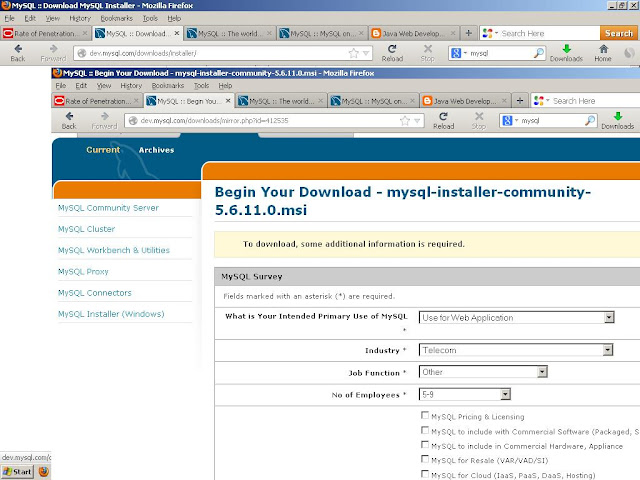Screenshot of a web browser window, specifically Firefox, capturing the process of downloading the MySQL installer. The Firefox logo is visible in the top-left corner, along with the browser title "MySQL - Download MySQL Installer - Mozilla Firefox." The image shows a cluttered interface with numerous open tabs. The primary tab displays a webpage titled "Begin Your Download - MySQL Installer Community 5.6.11.0.msi," which features a form that has popped up in front of other content. Another window with a similar heading, "MyInstallCommunity 5.6118," is also open. The webpage is segmented by a yellowish-orange divider, with the tab labeled "Current and Archives" highlighted in blue. The overall quality of the screenshot is low; it's slightly blurry and the elements appear small, making it difficult to discern details without context. The Windows Start button and the Firefox logo are also visible in the bottom-left corner of the screen.